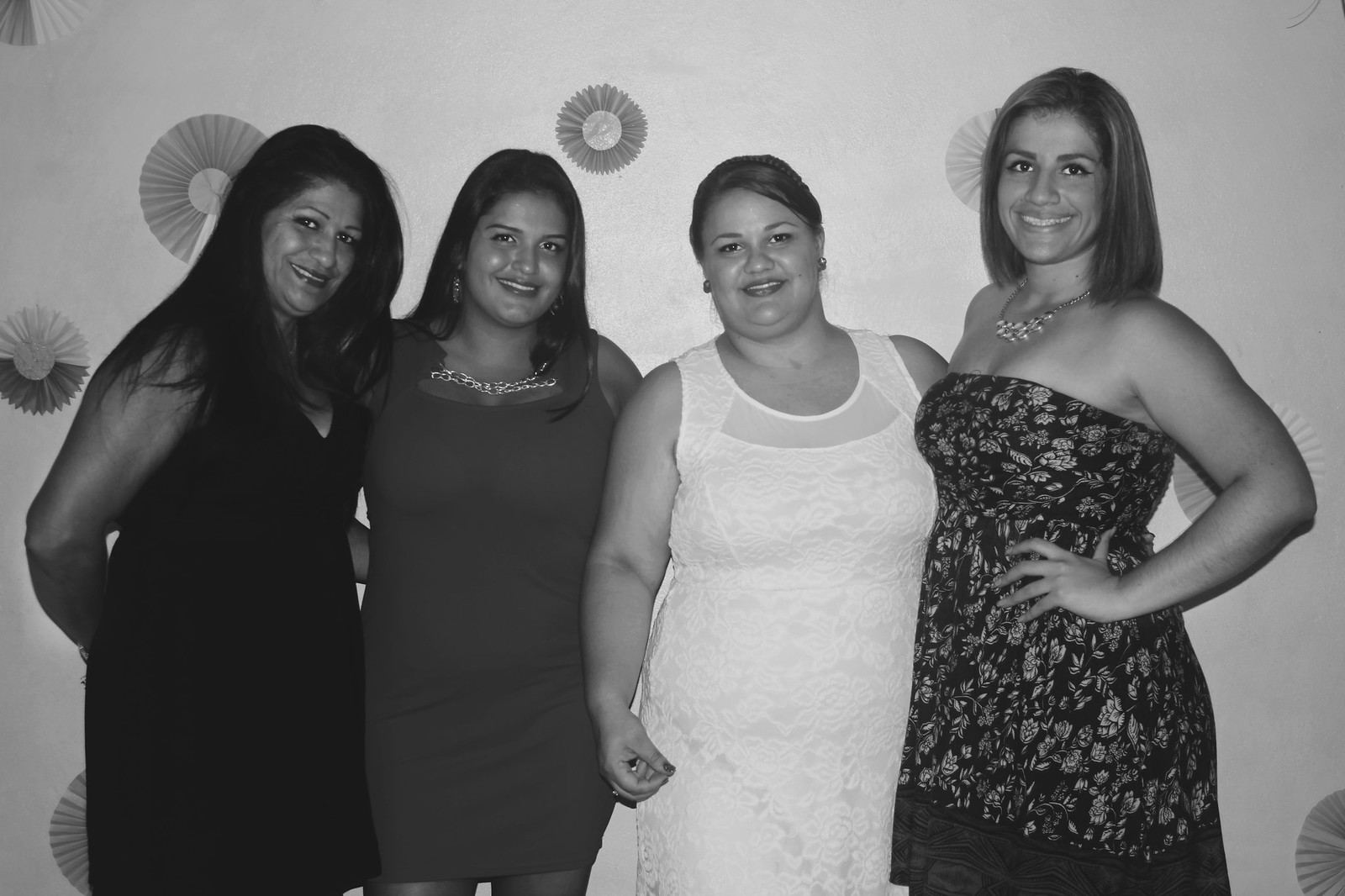In this black-and-white photograph, four women are posing together, smiling at the camera against a backdrop of a white wall adorned with circular decorations. The image captures them standing in a row, dressed in elegant attire that suggests they are attending a formal event, perhaps a party or a corporate function.

- The first woman, on the left, is wearing a v-neck, sleeveless dress.
- Next to her, the second woman is dressed in a sleeveless dress with a square neckline that falls to mid-calf.
- The third woman stands out with large earrings and a sleeveless white dress embellished with floral embroidery.
- The woman on the far right is in a strapless dress decorated with multiple flowers and accessorized with a white and gold necklace.

The entire photograph is slightly wider than it is tall, emphasizing the group’s elegant appearance and the setting, which, while monochrome, hints at a vibrant and celebratory atmosphere.